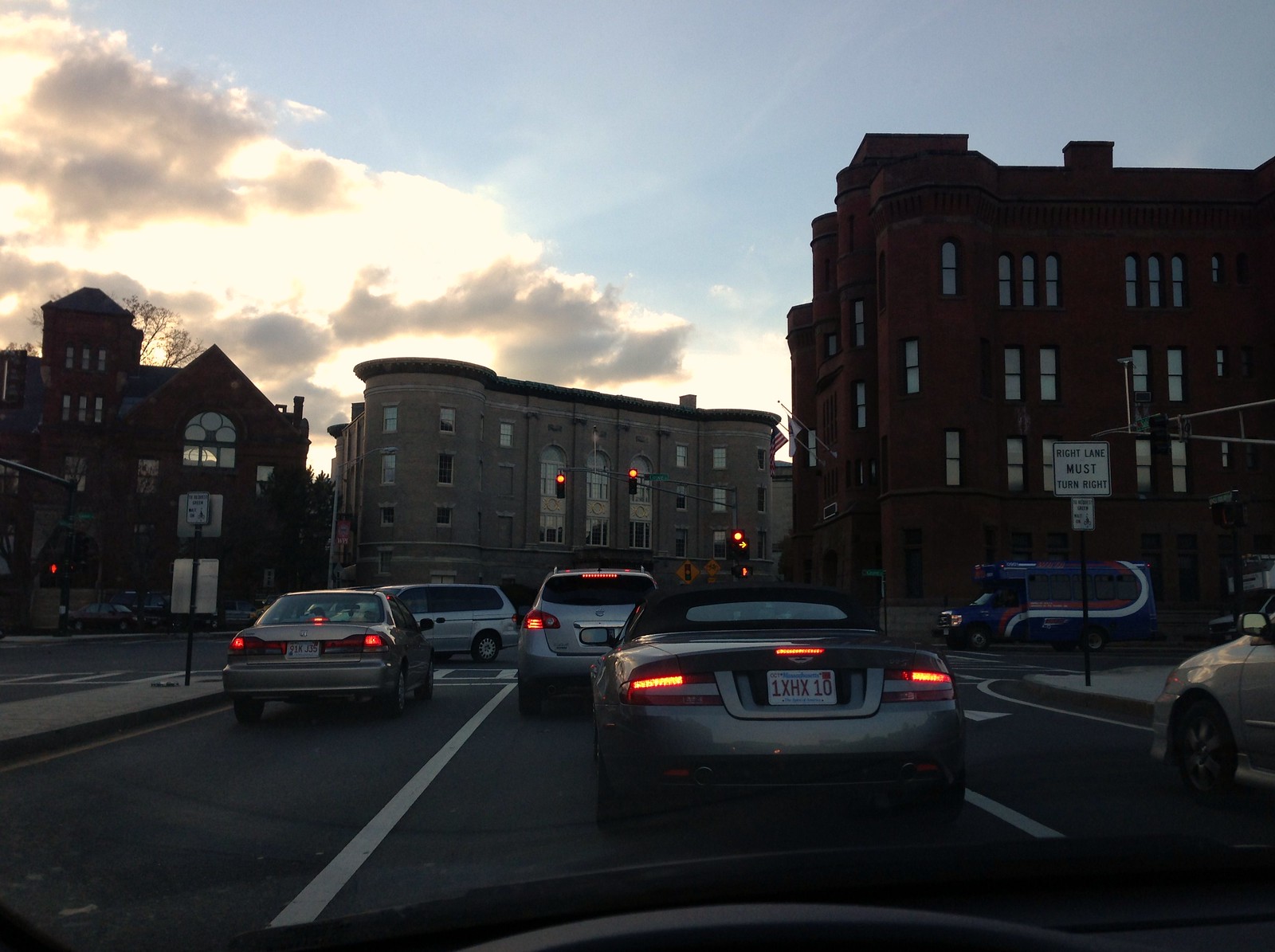This image captures a busy city intersection at dusk, viewed from inside a car stopped at a red traffic light. The sky is a light blue as the sun sets behind white clouds. Dominating the scene are the four-storey brick building on the right and another similar building straight ahead at the end of the street. The street is congested with cars, all displaying their red brake lights, including a sports car directly in front of the viewer's vehicle. A street sign indicating "Right Lane Must Turn Right" is clearly visible, and on this right lane, a distinctive blue van with a painted red and white line waits to turn at the T junction. To the right, parked in front of a large red brick building, is a small blue bus. On the left side of the intersection stands a large brick church, juxtaposed next to a light stone-colored building. The detailed elements of the cityscape and the warm hues of the setting sun create a vivid urban tableau.